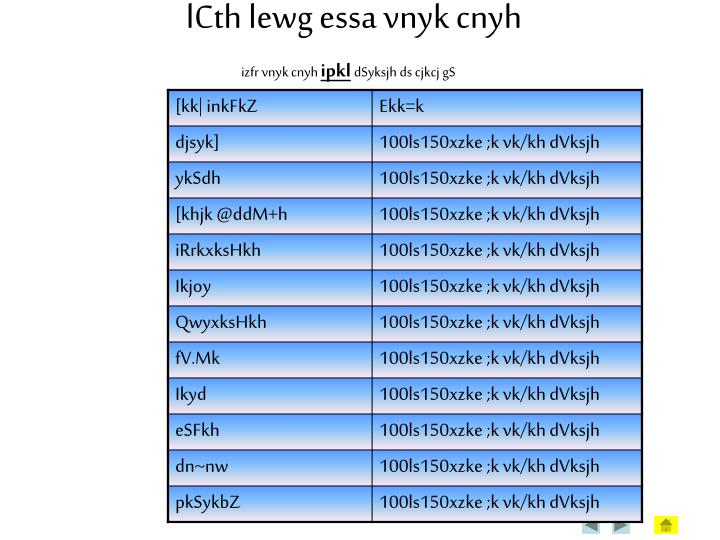The image displays a detailed, non-English table set against a blue background and bordered in black. At the top, in black text against a white background, it reads "ekvleguesa vinyksynta." Below this, there is bolded and underlined text reading "IPKL," followed by additional, similarly styled writing. The table is divided into around 12 rows and two columns by blue lines. The left column contains shorter entries, primarily consisting of a word or phrase with both letters and numbers, while the right column features more extensive text combinations, again primarily with letters and numbers. The top entry in the right column uniquely states "ekk equals k," while subsequent entries include various numeric and alphanumeric codes such as 100, ls, 150, x, z, ke, and others. The distinctive presentation and formatting imply a structured explanation or categorization, despite the cryptic nature of the text.